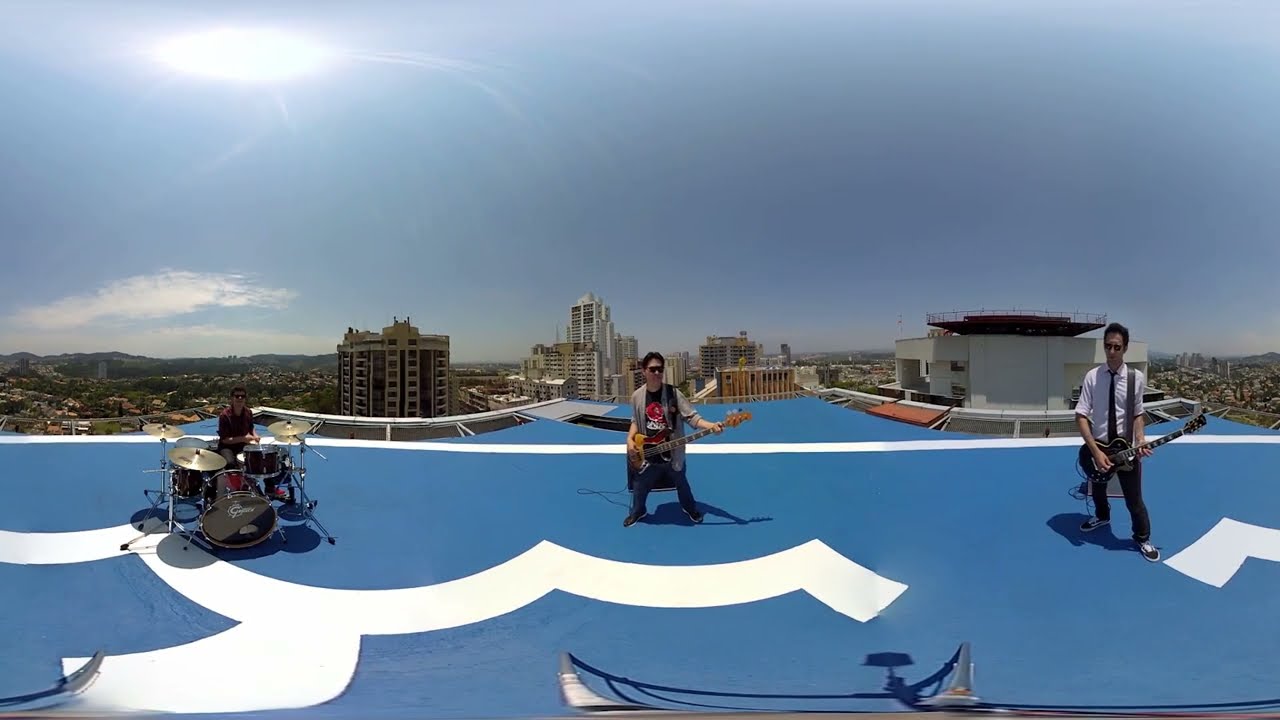In this detailed promotional photograph, a three-piece band is positioned on a blue-painted rooftop with white markings. The cloudy gray sky above and the distant cityscape with tall buildings provide a striking backdrop. The scene is as follows:

On the left side, the drummer sits behind his kit, partially obscured by shadow but distinguishable by his red-sleeved shirt. The cymbals are prominently placed in front of him. In the center stands a bassist, head tilted to the left, donning sunglasses and a gray trench coat while gripping his bass guitar. To the right, another guitarist stands, also wearing sunglasses. He sports a light-colored shirt with a suit and tie, paired with black pants and tennis shoes with white laces. Each guitarist has an amp situated behind them.

The towering city skyline includes a mix of buildings: a tall gray structure with a lighter gray top on the left, a white building towards the center, and a white-walled stadium with a red section and barrier on the far right. The scene is lit by a faint pinkish glow in the upper left corner, suggesting sunshine attempting to break through the clouds, enhancing the overall aesthetic of this elevated rooftop stage.